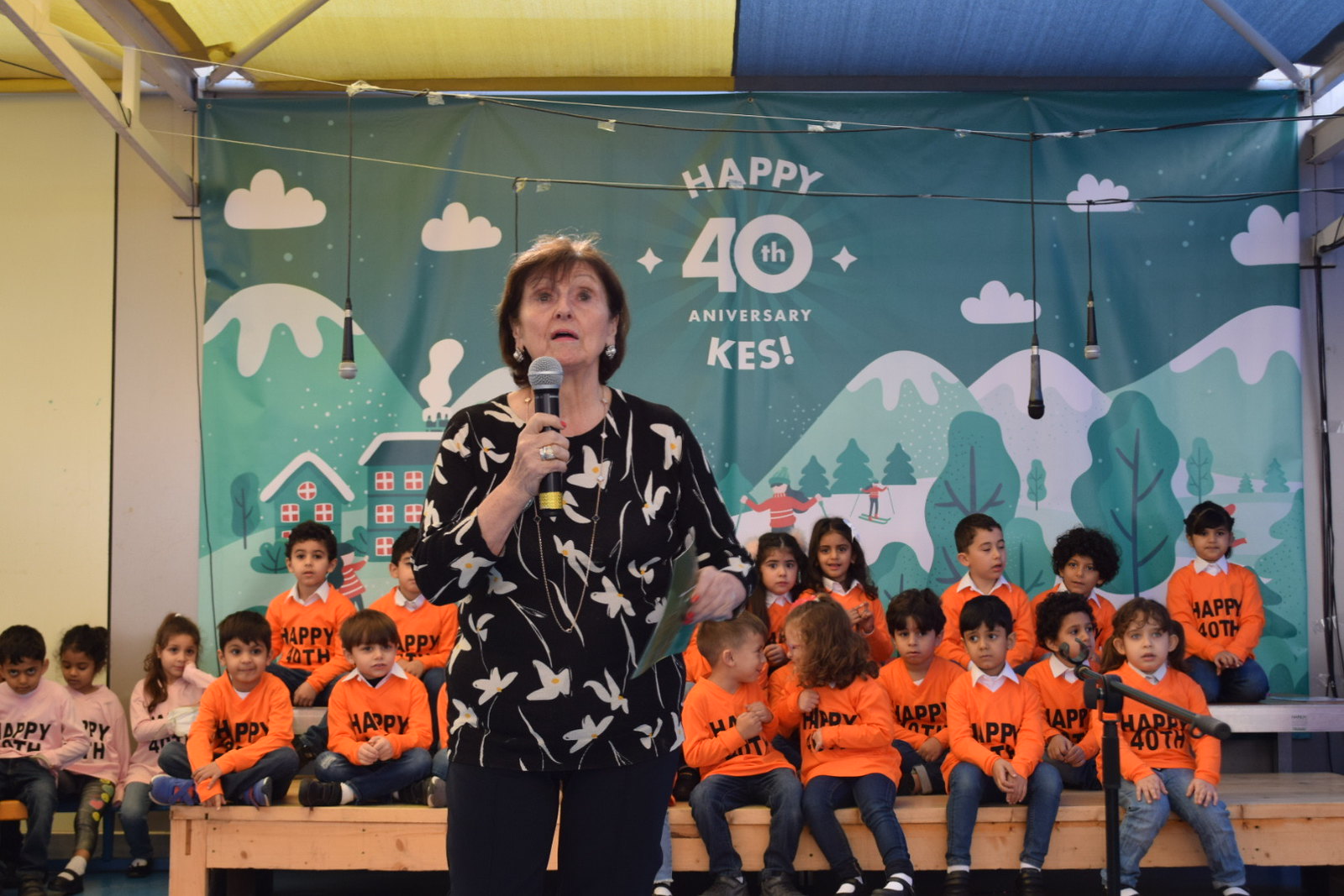The image captures a lively scene where an older white woman with brown hair, dressed in a black long-sleeve shirt adorned with white flowers and black pants, is standing and speaking into a microphone. She gestures with her left hand, which holds a pamphlet, while a ring glistens on her right ring finger. The backdrop features a large banner reading "Happy 40th Anniversary KES," illustrated with images of mountains, skiers, and trees. Seated on wooden and metal bleachers behind her are approximately 20 children, divided into two groups wearing either long-sleeve orange or pink shirts with the same "Happy 40th" text. The gymnasium setting is filled with the natural vibrancy of children, some of whom are seen laughing, misbehaving, and interacting joyfully with one another.